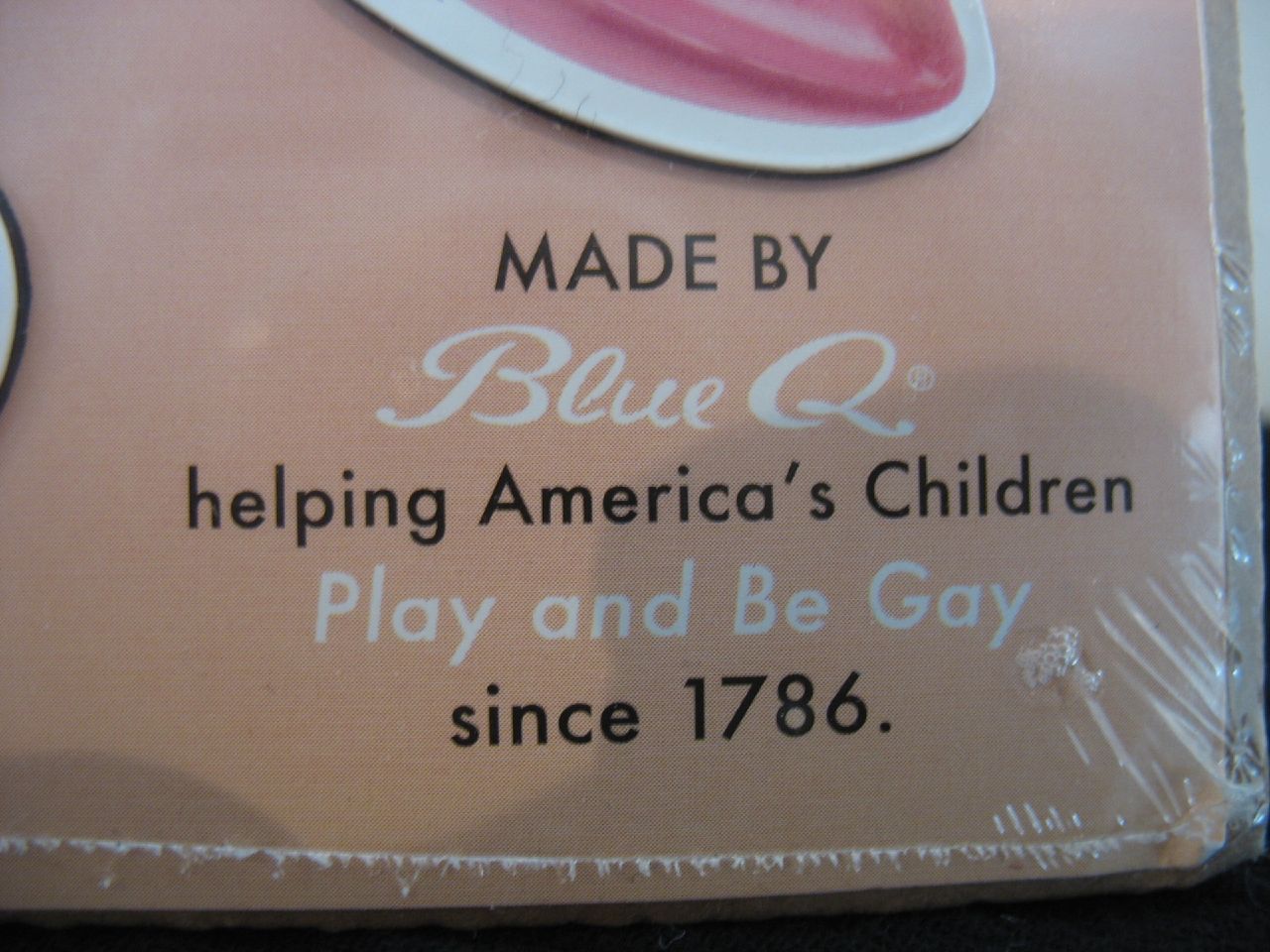The image features a product wrapped in tight, slightly reflective plastic packaging. The packaging displays various texts and elements. At the top, there is a pink detail, bordered by white edges. Below, in black text, the words "Made by" are written, followed by "Blue Cube" in white text. Continuing down, "Help in America's Children" is printed in black text, followed by "Play and Be Gay" in white text. Finally, "Since 1786" is in black text at the bottom. The background appears to be brown fabric visible through the plastic. The packaging is drawn tightly, particularly on the right side, revealing the edges at the bottom.